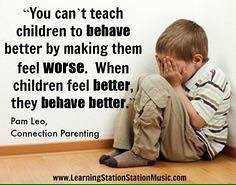The image depicts a somber scene of a young boy sitting forlornly in the corner of a room. He is dressed in a white polo shirt adorned with brown and green stripes and brown khaki pants. His socks are a similar earthy hue. The boy is curled up with his legs bent, burying his face in his hands, conveying a sense of sadness or distress. The room is minimally decorated with white walls and a brown wooden floor, contributing to the overall feeling of isolation.

Prominent text overlays the image, delivering an important message: "You can't teach children to behave better by making them feel worse. When children feel better, they behave better." This message is attributed to Pam Leo, a notable figure in Connection Parenting. The advertisement aims to promote compassionate and effective parenting techniques, urging viewers to visit the website www.learningstationmusic.com for more information. The overall tone and presentation of the image suggest a call to end harsh disciplinary practices and encourage kinder, more supportive parenting methods.